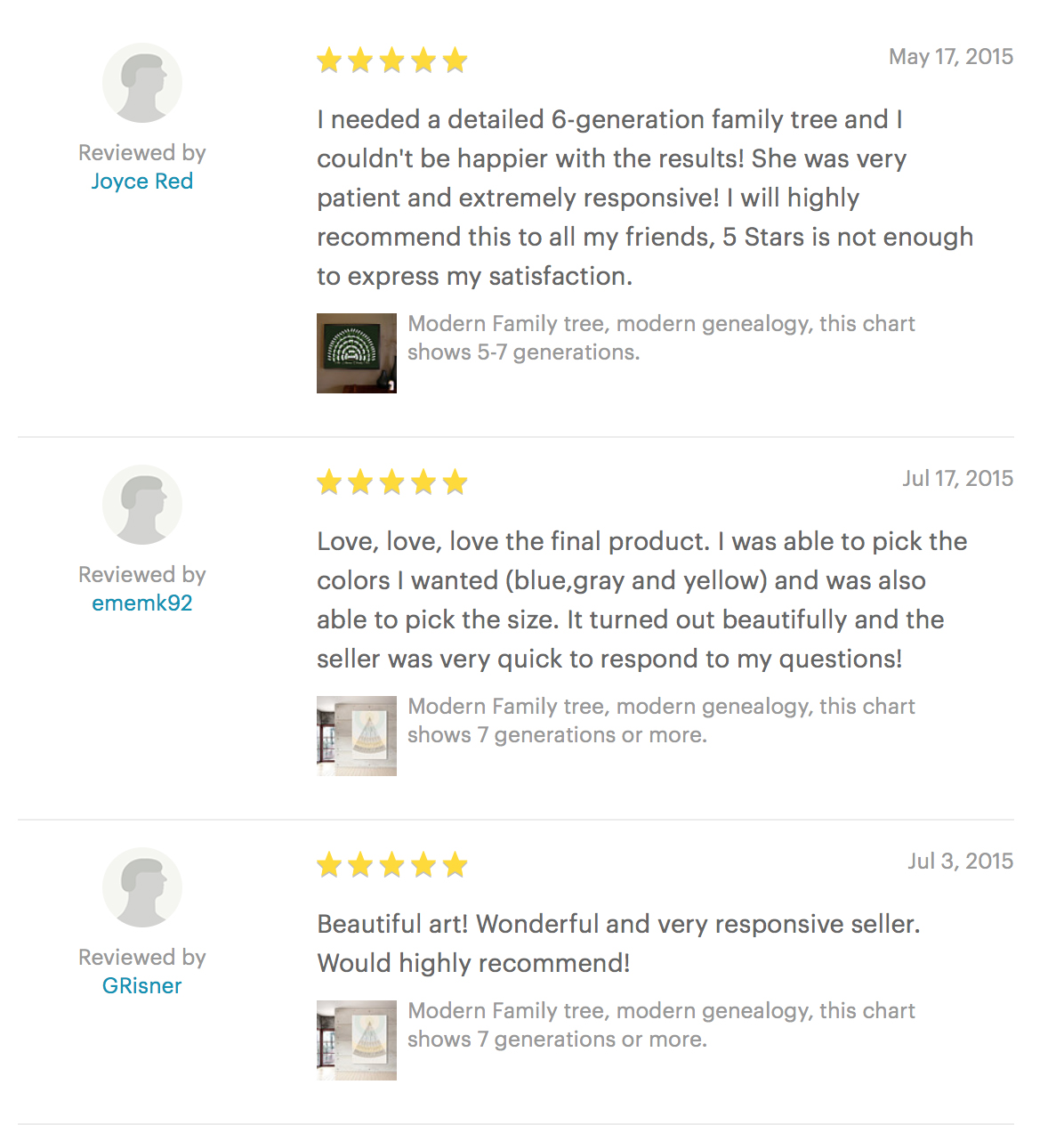Here is a cleaned-up and detailed caption for the described image:

---

The image features a clean white background with a circular design on the left-hand side, containing a gray circle. Within the circle, text reads "Review" and "Buy" in gray, while inside a blue circle, it says "Choice" and "Read" in red. Below this, five gold stars are displayed alongside black text stating, "I needed a detailed six-generation family tree, and I couldn't be happier with the results. She was very patient and extremely responsive. I would highly recommend this to all my friends. Five stars is not enough to express my satisfaction." This review endorses "Modern Family Tree, Modern Genealogy," and it specifies that the chart shows five to seven generations, posted on May 17, 2005.

The next review begins similarly with "Review" and "Buy" in gray, followed by a blue circle with text reading "E-M-E-M-K-92." It is rated five stars and says, "Love, Love, Love the final product. I was able to pick the colors I wanted (blue, gray, and yellow) and also the size. It turned out beautifully, and the seller was very quick to respond to my questions." The review also promotes "Modern Family Tree, Modern Genealogy," indicating this chart shows seven generations or more.

The final review again starts with "Review" and "Buy" in gray, and a blue circle containing "G-R-I-S-N-E-R." It gives five stars and exclaims, "Beautiful Art! Wonderful and responsive seller, would highly recommend." This review praises "Modern Family Tree, Modern Genealogy," mentioning that the chart displays seven generations or more. It was posted on July 3, 2015.

Each review is separated by thin gray lines for clarity.

---

This caption provides a clear and thorough description of the image content, preserving all the details mentioned in the original summary.